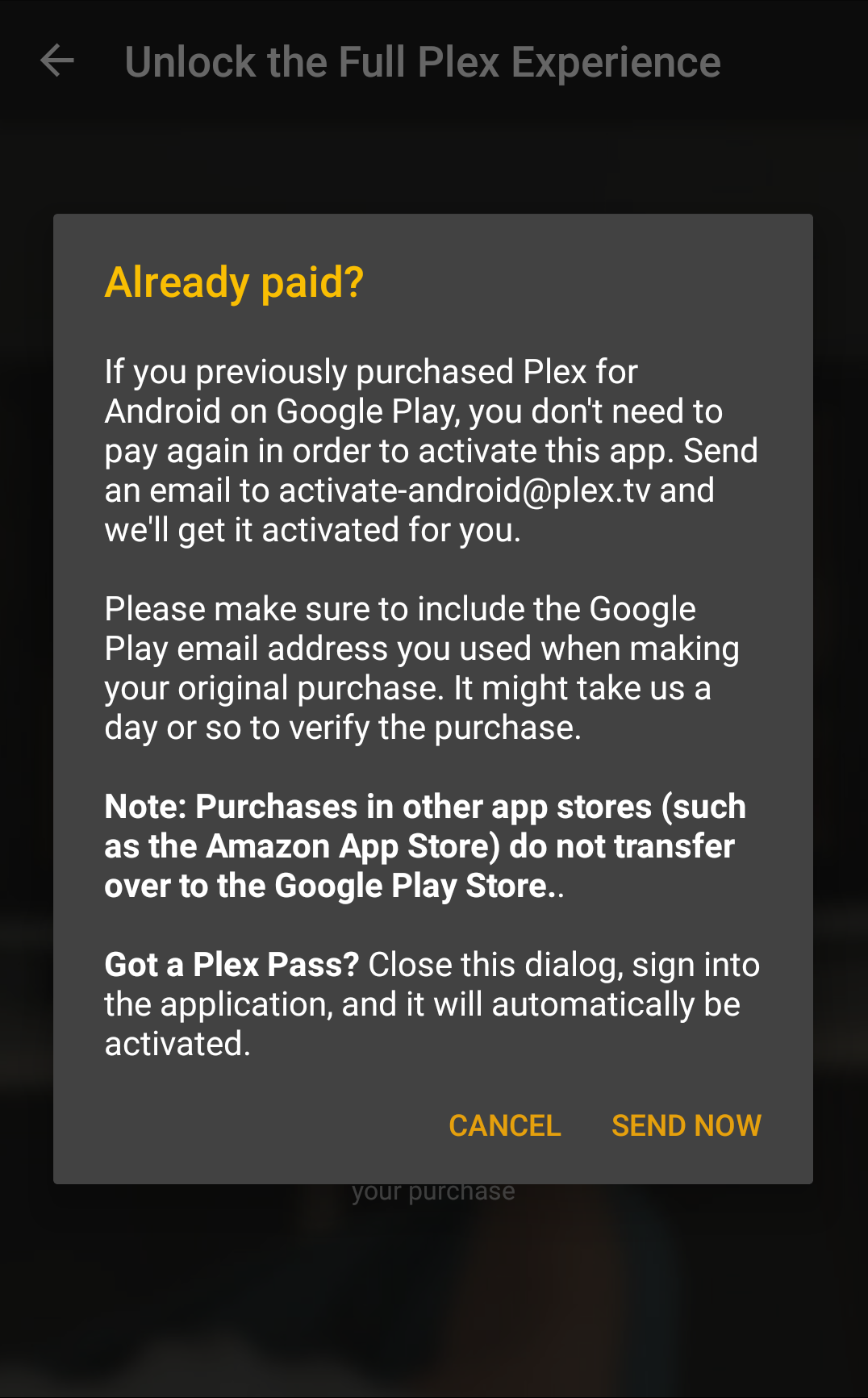The image features a vertically rectangular frame. The main window is predominantly black, and a dark gray pop-up window overlays it. At the top of the main background, the text reads "Unlock the full Plex experience." 

Within the pop-up window, the top left corner displays a yellow banner with the text "Already paid?" in white letters. Below this, it states in white text: "If you previously purchased Plex for Android on Google Play, you don't need to pay again to activate this app. Send an email to activate-android@plex.tv, and we'll get it activated for you. Please make sure to include the Google Play email address you used when making your original purchase. It might take us a day or so to verify the purchase." 

In bold white text, it notes: "Purchases in other app stores such as the Amazon App Store do not transfer over to the Google Play Store."

Beneath that, in bold text, it asks: "Got a Plex Pass?" Following this is an instruction in regular white text: "Close this dialog, sign into the application, and it will automatically be activated."

At the bottom right corner of the pop-up window, there are two buttons labeled "Cancel" and "Send Now."